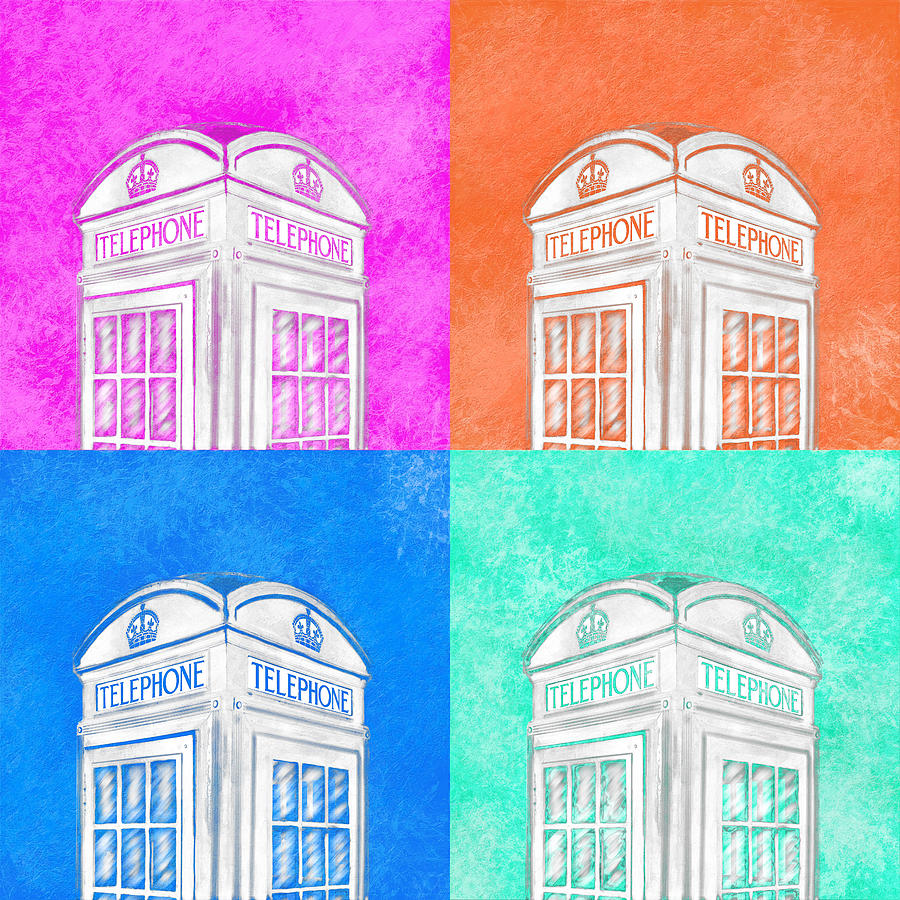This illustration features a quartet of British-style iconic phone booths, each rendered in a distinct color scheme. The topmost phone booth is set against a vivid magenta backdrop, with a magenta crown and the word "telephone" inscribed in matching magenta hues. The booth itself remains predominantly white, accented by magenta details, including its outlined door.

Below this, the next phone booth is immersed in a vibrant blue background. The crown and the word "telephone" on this booth are presented in the same bright blue. Like the others, the booth's body stays white, with the door outlined in blue, seamlessly blending into its colorful surroundings.

Next is a phone booth engulfed by an energizing orange background, consistent with the previous designs. The orange crown and the inscription "telephone" follow suit, set upon the crisp white booth, whose door is meticulously outlined in orange.

The final phone booth stands out with its cool aqua theme. An aqua background, crown, and "telephone" label adorn the otherwise white booth, maintaining the design's coherence by outlining the door in aqua.

Throughout the image, the backgrounds sport a sponge-paint texture, enriched with subtle white shadings that add depth and dimension to the entire scene. This artistic touch enhances the vibrancy and visual appeal of the classic British phone booths.